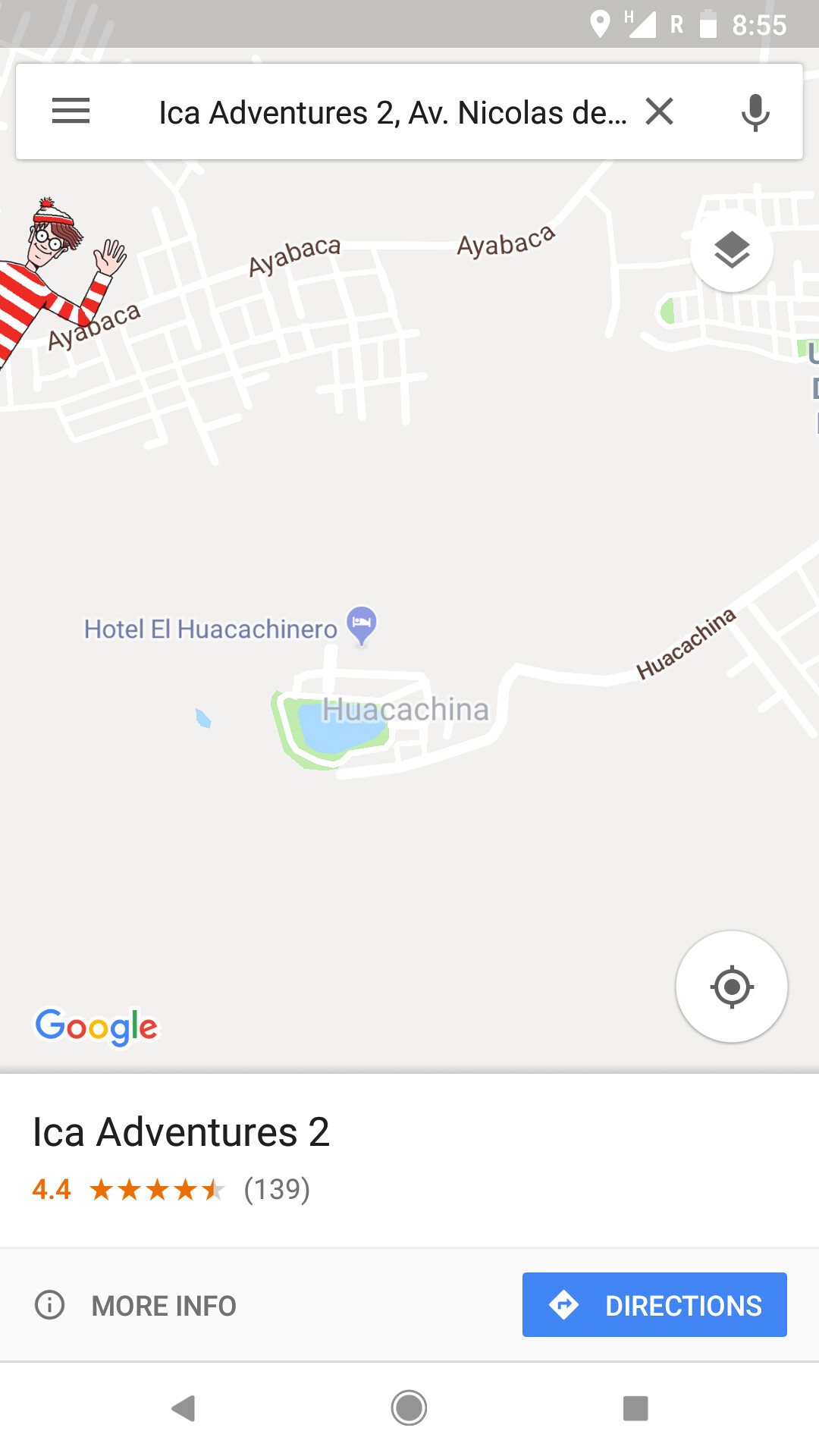The image depicts a Google Maps screen. At the very top, there is a gray status bar that includes various cell phone icons on the right, such as the current time, battery percentage, and "A55." Directly below the status bar is the search bar where the query "ICAadventures2, av. nicolasde..." is partially visible. 

Beneath the search bar, the main map section is displayed. In the top-left corner of the map, a "Where's Waldo" icon appears, with Waldo waving his right hand. Along the top edge of the map, part of the street name "AYABACA" is visible. 

Towards the bottom of the map section, a hotel icon labeled "HUACAChina" is present. The background of the entire map area features a subtle gray tone.

Further down, just below the map, there is an entry for "ICAadventures2" with a 4.4 rating indicated by four and a half orange stars and 139 reviews. Beneath this rating, there are two prominent buttons: a "More Info" icon on the left and a blue "Directions" button on the right.